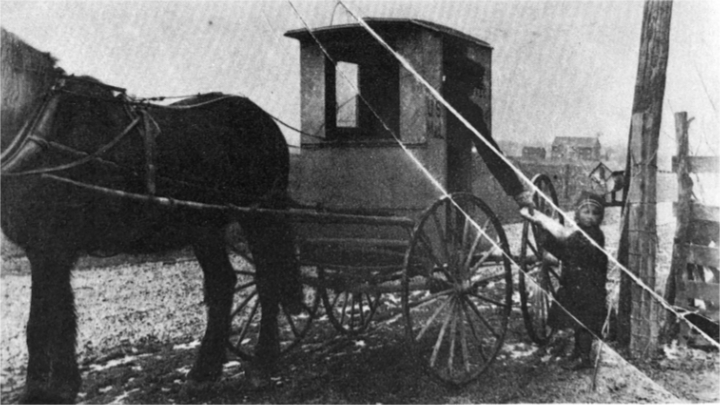In this black-and-white photograph, an era long past comes to life as a solitary, strong horse draws an old-fashioned mail carriage with four slender-spoked wheels. The carriage, emblazoned with "US Mail" on its side, stands motionless on a dirt road. A telephone pole rises on the right, its lines either climbing into the sky or marking the photograph's age through weathering. A small child, dressed in dark clothing and wearing a hat, stands beside the carriage, extending a hand to receive a letter from a barely discernible mail carrier within the carriage. The carrier, almost lost in shadow, reaches out through an open window, connecting the past with the moment. Behind the child, a lone tree stands sentinel, while the faint outline of a homestead or house forms the distant backdrop, giving context to this poignant scene of early mail delivery.